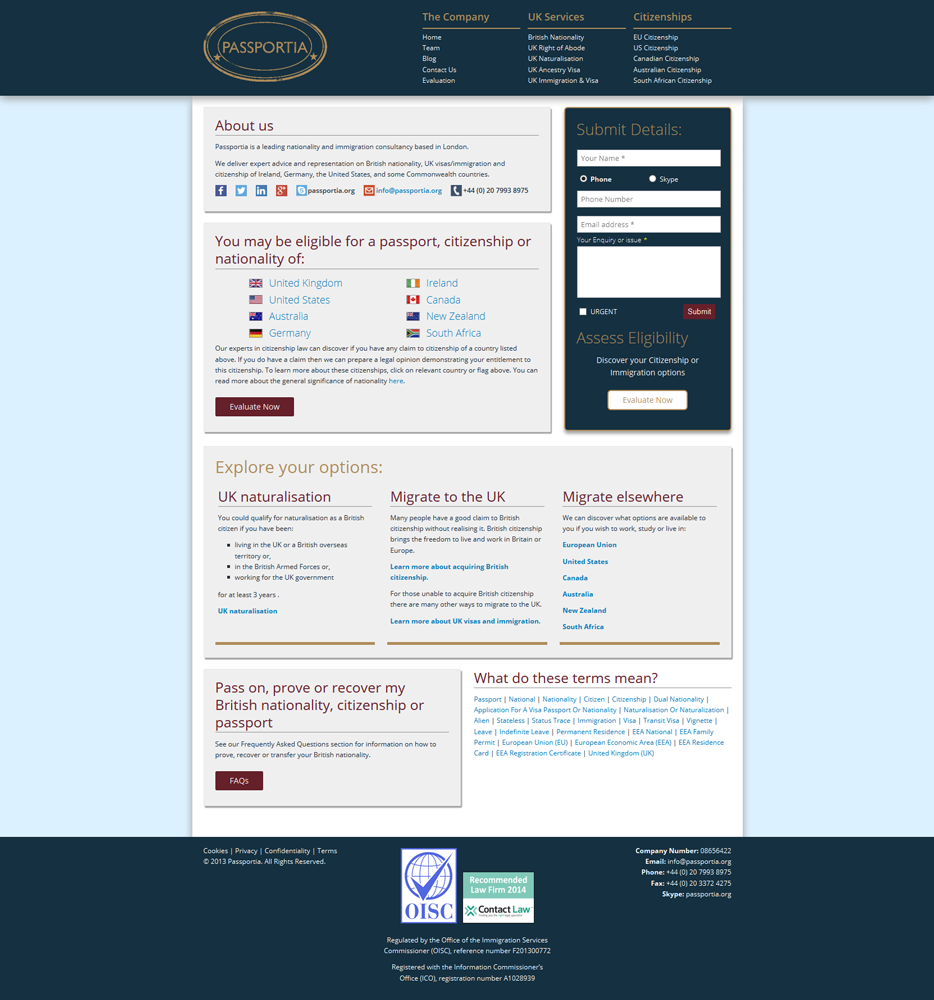**Caption:**

The image features a sleek, black background with an orange circle slightly right of the center. Inside this circle, the text "Casa Porta" is prominent. To the far right at the top, the company's services are listed underlined in orange: "UK Services," "Citizens," and "Citizenships."

Beneath these headings, there are clickable white text buttons. Under "UK Services," you find: "Home," "Team," "Blog," and "Contact Self-Evaluation." Similarly, under "Citizens," options include: "British Nationality," "UK Right of Adobe," "UK Naturalization," "UK Ancestry Visa," "UK Immigration," and "Visa." Lastly, under "Citizenships," the options are: "EU Citizenship," "US Citizenship," "Canadian Citizenship," "Australian Citizenship," and "South African Citizenship."

Further down, the left and right sections have grey backgrounds with white inner boxes. The left side contains multiple grey boxes. The first box has "About Us" with a detailed description. Below is a section that suggests eligibility for passports, citizenships, or nationalities in highlighted blue text, including countries like the United Kingdom, United States, Australia, Germany, Ireland, Canada, New Zealand, and South Africa, followed by additional black text.

On the upper right side, there is a black background with white text fields for user information such as name, phone number, email address, and inquiry details. There's also a green-texted section labeled "Support Your Options," followed by bullet points like "UK Naturalization," "Immigrate to the UK," and "Immigrate Elsewhere."

Finally, at the bottom, a blue background features white text with contact information including phone numbers, fax numbers, and a copyright date.